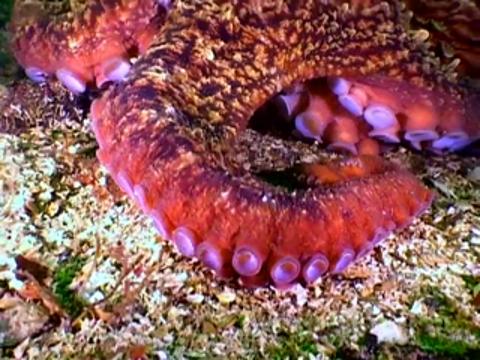The image depicts a vibrant underwater scene featuring what appears to be the tentacle of an octopus. The tentacle is primarily red with light pink and purple circular suction cups, giving it a rough appearance and almost glowing or neon quality. It seems to be swirled and curled, with multiple tentacles visible—one prominently in the center, another in the upper left corner, and a third in the upper right corner. The background appears to be a rocky or pebbly surface in shades of green, white, and light tan, possibly resembling a mossy underwater terrain. The upper part of the tentacle displays a beige-brown speckled pattern, while the sides are more vividly red and purple. The photo is taken close up, making it difficult to discern the exact environment but suggesting an underwater setting due to the color and texture details.